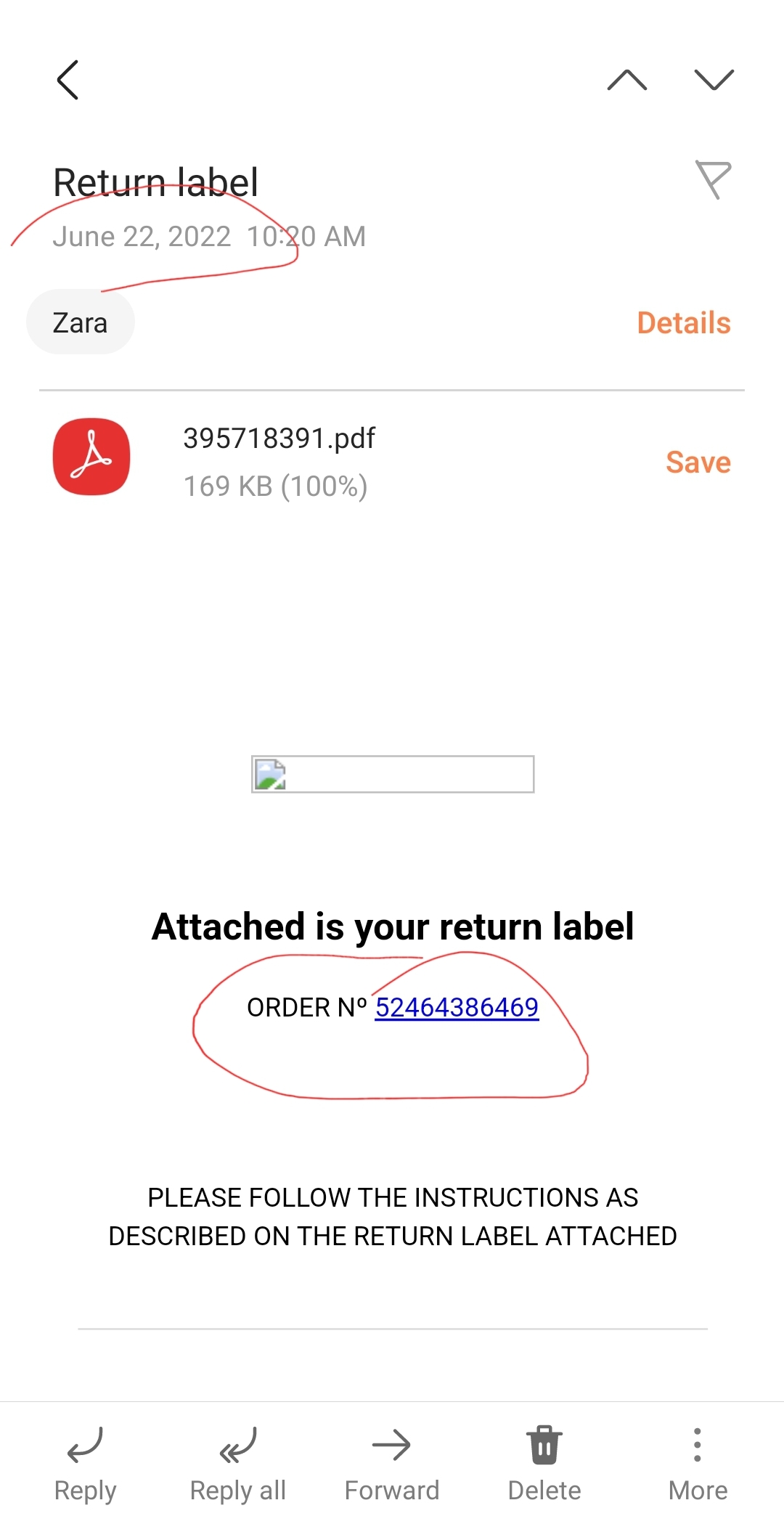The image depicts a white screen displaying an email on which specific elements have been marked. At the top of the screen, the text reads "Return Label June 22, 2022," which is circled in red with a thin, irregular line. Below this, the timestamp "10:20 a.m." is visible, followed by the brand name "Zara." To the right of "Zara," the word "Details" appears in orange.

A horizontal line separates the upper text from a section in the middle of the screen where a PDF logo is visible. The logo, depicted in red with a swirly triangle design, is accompanied by the filename "395718391.pdf (169 KB, 100%)." To the right of the PDF information, the word "Save" is highlighted in orange, suggesting a clickable option.

Below this, there seems to be a search bar with a broken image icon. Further down, text instructs, "Attached to your return label order number 52464386469," with the order number circled in red similarly to the date mentioned above. In black text beneath this, it reads, "Please follow the instructions as described on the return label attached."

At the very bottom of the screen, typical email action options are visible, including "Reply," "Reply All," "Forward," "Delete," and "More." There are also two horizontal lines that visually separate different sections of the email interface. This structured layout strongly suggests that the image is a screenshot of an email, particularly one concerning a return label from Zara.